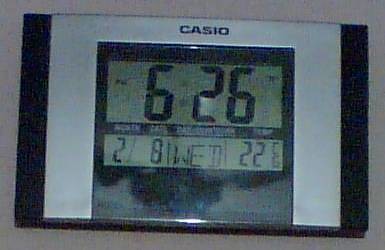This image features a compact, rectangular Casio digital clock prominently displaying the time, 6:26 PM, on a dull green digital screen interface. Nestled on a white background, the clock's composition includes a silver body with black borders on the left and right edges. The top of the clock boasts the brand name "Casio" in reflective silver lettering. Below this, the digital display houses several smaller rectangles showing additional information: the date (February 8th, marked as "2-8"), the day (Wednesday, abbreviated as "WED"), and the temperature (22 degrees Celsius). Despite its small size, the clock's layout and contrasting black text on a green screen convey the essential details clearly. The image is captured indoors, seemingly under natural lighting.